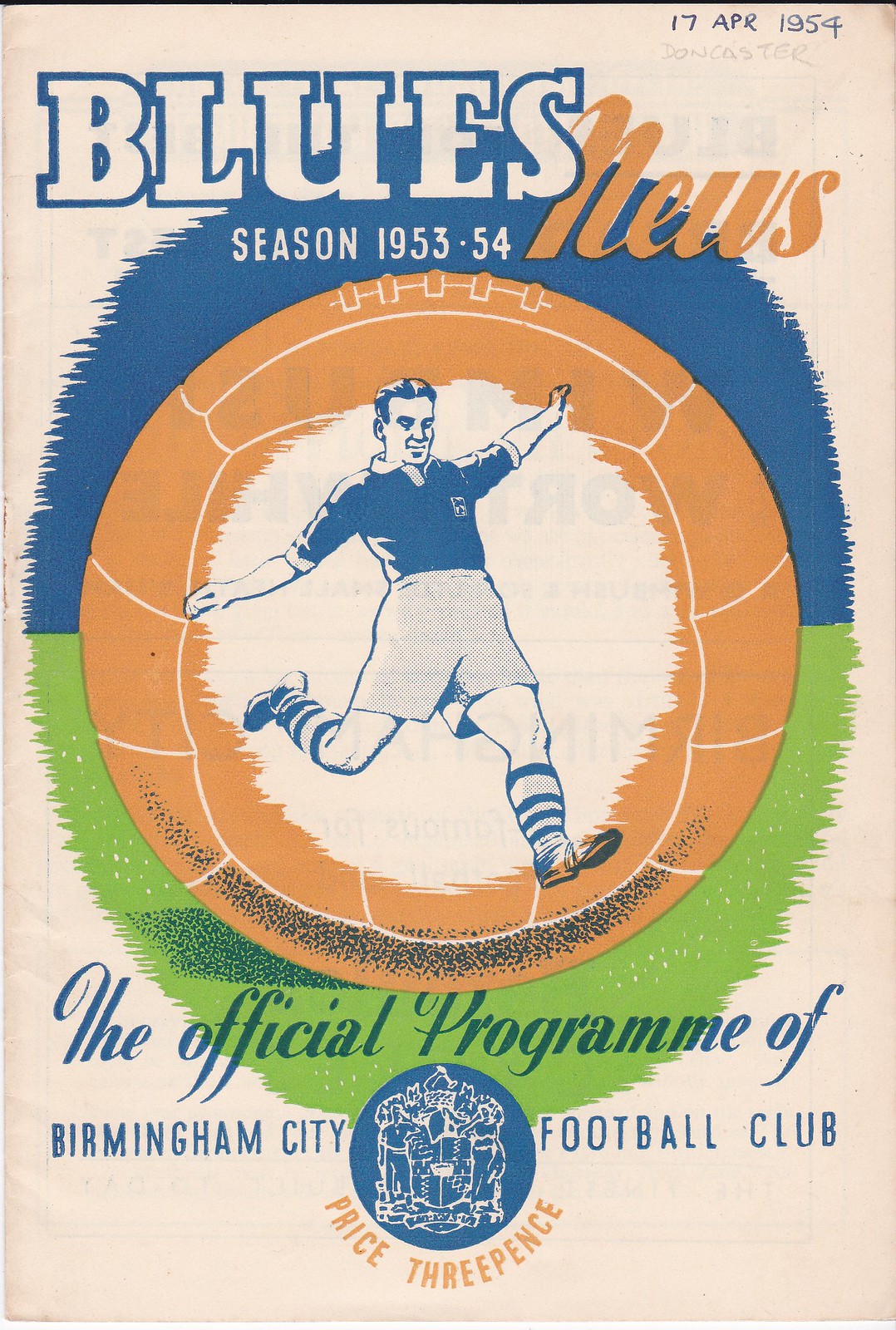The image depicts an old football club program dated April 17, 1954. Featured prominently in the center is a drawing of a football player poised to kick a ball, intriguingly illustrated as if he is inside a large soccer ball. The program is titled "Blues News Season 1953-54" and is identified as the official program of Birmingham City Football Club. The cover also displays a logo, though its details are somewhat hard to discern. At the bottom, it notes the price, which is 3 pence. The entire image, rendered clearly and vividly, includes a range of colors from blue to green to orange.